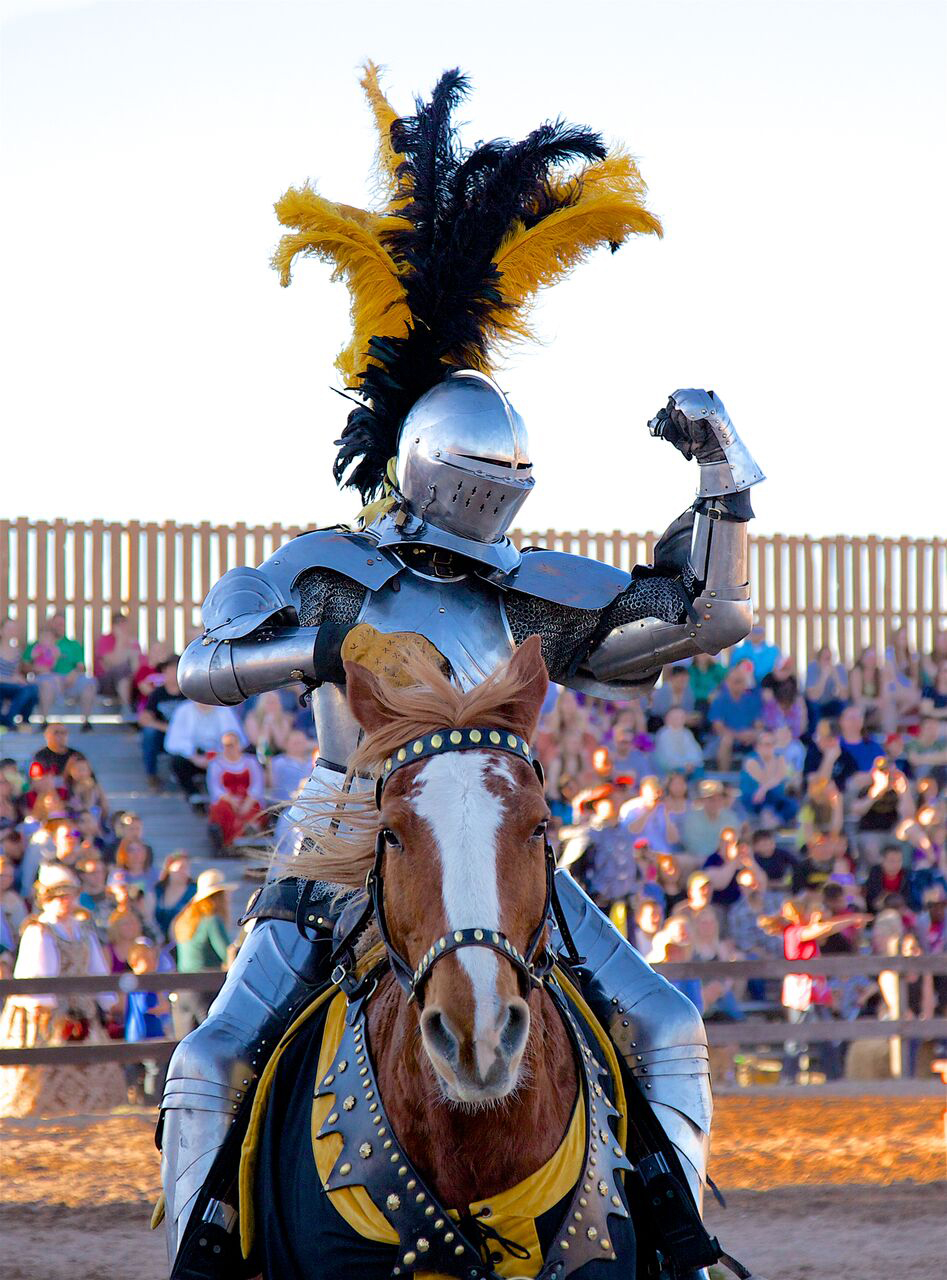In the image, a knight in full silver metal armor sits atop a brown and white horse adorned in blue and yellow gear. The knight's armor includes intricate chainmail underneath, and his helmet boasts a striking plume of blue and yellow feathers. He raises his right arm in a celebratory or flexing gesture. The horse, similarly decked out in matching blue and yellow attire, has a sash wrapped around its neck. They appear to be part of an outdoor event, likely a modern fair, with an audience seated behind a series of fences or bleachers. The audience is casually dressed, and the background is slightly blurred, but you can see a large, towering wooden fence enclosing the area. The setting is outdoors under the bright daytime sun, adding to the vibrant atmosphere of the gathering.